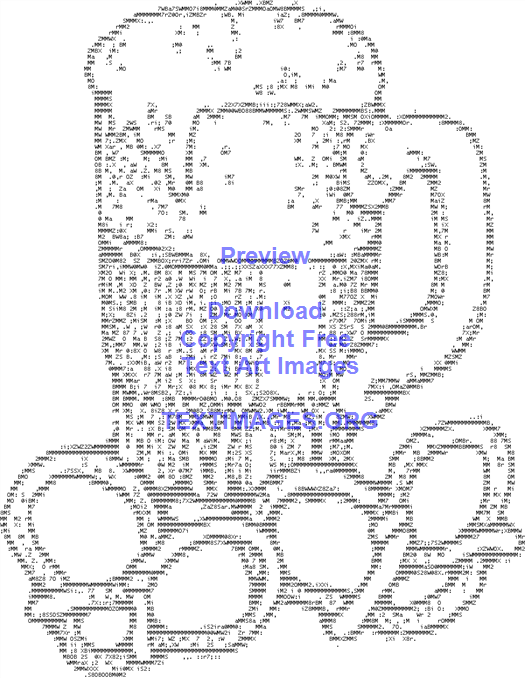The image showcases a striking piece of text art, where carefully arranged letters, numbers, and various keyboard characters form an authentic-looking glass mug of beer. The mug, frosty at the top with foam overflowing down the sides, is accompanied by two pretzels in the foreground, each approximately the same size as the mug's handle. The entire composition, apart from a watermark in blue or purple font, is rendered in black and white. The watermark reads, "Preview. Download copyright-free text art images at textimages.org." The intricate details and lifelike representation make this a captivating and realistic example of text art.